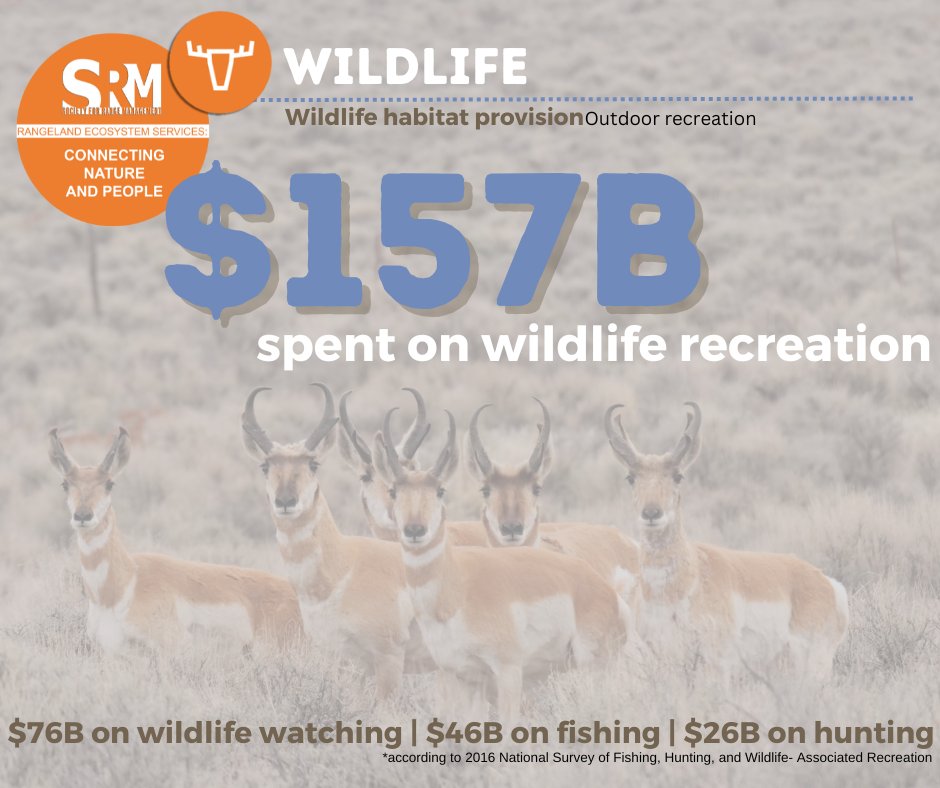The image is a detailed informational poster from Strangeland Ecosystem Services (SRM), promoting the connection between nature and people. The poster features a gray background with a faded picture of six deer standing in a grassland area. Prominently displayed at the top, it reads "Wildlife Habitat Provision, Outdoor Recreation," highlighting that $157 billion is spent on wildlife recreation. Key figures from the 2016 National Survey of Fishing, Hunting, and Wildlife-Associated Recreation are also cited, noting $76 billion spent on wildlife watching, $46 billion on fishing, and $26 billion on hunting. The upper right corner of the poster features the SRM logo, an orange circle containing an outline of a deer head, along with the tagline "Connecting Nature and People." Some text details in the image are highlighted in blue with a subtle shadow effect, adding emphasis to the financial statistics presented.